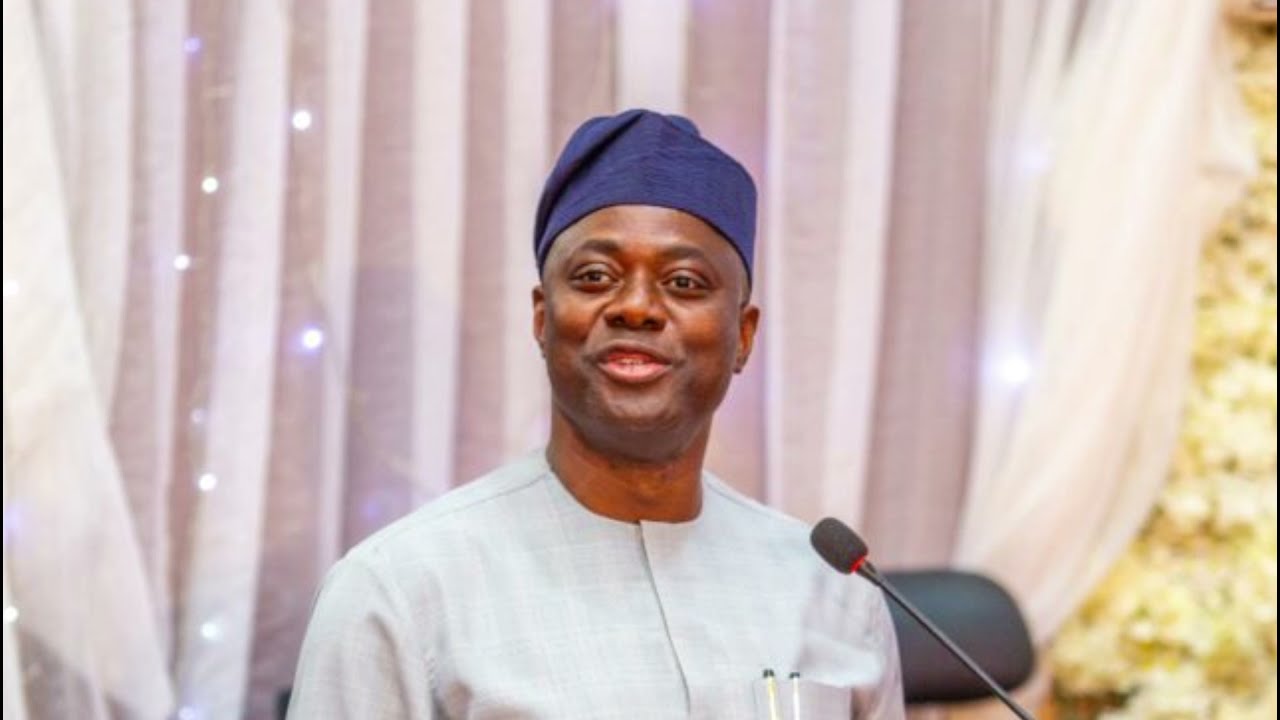In the center of the image stands a black man wearing a blue African-style cap, which fits snugly on his head. He is donning a bluish-white, long-sleeve, button-down shirt with two pens visibly clipped into the left breast pocket. The shirt is buttoned all the way to the top, featuring a circular-color neckline. The man, who has a slight five o'clock shadow, is smiling warmly as he looks straight ahead. Positioned in front of him at chest level is a microphone, suggesting he is either about to speak or in the middle of a conversation.

The background features a sheer, white pleated curtain adorned with a few twinkling, sparkly lights, possibly indicating a festive setting. To the right of the curtain, a grainy, yellowish element ascends from the bottom of the frame, which one caption suggests might resemble a goldish tree or Christmas decoration. The curtain's translucency and light dispersion add an atmospheric touch to the photograph. Additionally, there is a chair visible behind him on the left side, albeit unoccupied. The overall setting is indeterminate, giving no clear indication of whether the scene occurs indoors or outdoors.